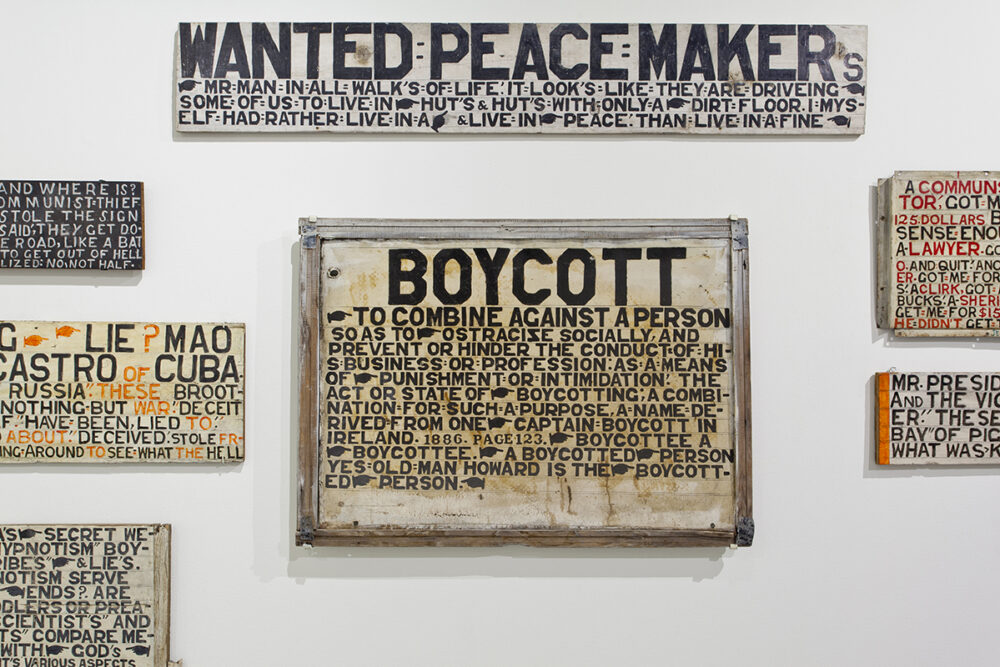This photograph, taken indoors against a light gray wall, features an array of old wooden signs with various inscriptions. At the center top, a long horizontal sign with bold black print reads, "Wanted Peacemaker," followed by smaller text: "Mr. Man in all walks of life. It looks like they are driving some of us to live in huts with only a dirt floor. I myself had rather live in peace than in a fine." Below this, there is another slightly rectangular wooden sign outlined in a light wood color, boldly captioned "Boycott." The detailed text defines the term: "To combine against a person so as to ostracize socially and prevent or hinder the conduct of his business or profession as a means of punishment or intimidation, the act or state of boycotting in combination for such a purpose, a name derived from one Captain Boycott in Ireland. Boycottee, a boycotted person. Yes, old man Howard is the boycotted person." The photograph also shows five additional signs—three on the left and two on the right—though they are partially cut off and their contents are hard to read. The overall dimensions of the photograph are approximately six inches wide and four inches high.